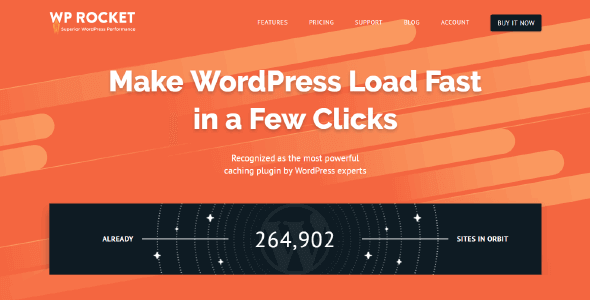The image depicts a website with a vivid orange background adorned with lighter orange horizontal stripes running across it. At the top left corner, the text "WP Rocket" is prominently displayed in white. Positioned towards the top right are navigational links labeled "Features," "Pricing," "Support," "Blog," and "Account." Below these links, a black rectangular button with white text states "Buy It Now."

Centrally located on the page, large white text proclaims, "Make WordPress Load Fast," with a sub-line underneath that reads, "in a few clicks." Beneath this, in smaller white font, the text declares, "Recognized as the Most Powerful Caching Plugin by WordPress Experts," with "Caching" phonetically spelled out in parentheses.

A large, elongated black rectangle spans the width of the page, featuring a distinctive, radar-like circular design on either side. On the left side of this rectangle, a vertical white line indicates the text "All Ready." In the center, a numerical figure "264,902" is prominently displayed, followed by another vertical white line on the right accompanied by the words "Sites in Orbit," completing the detailed and structured layout of this image.